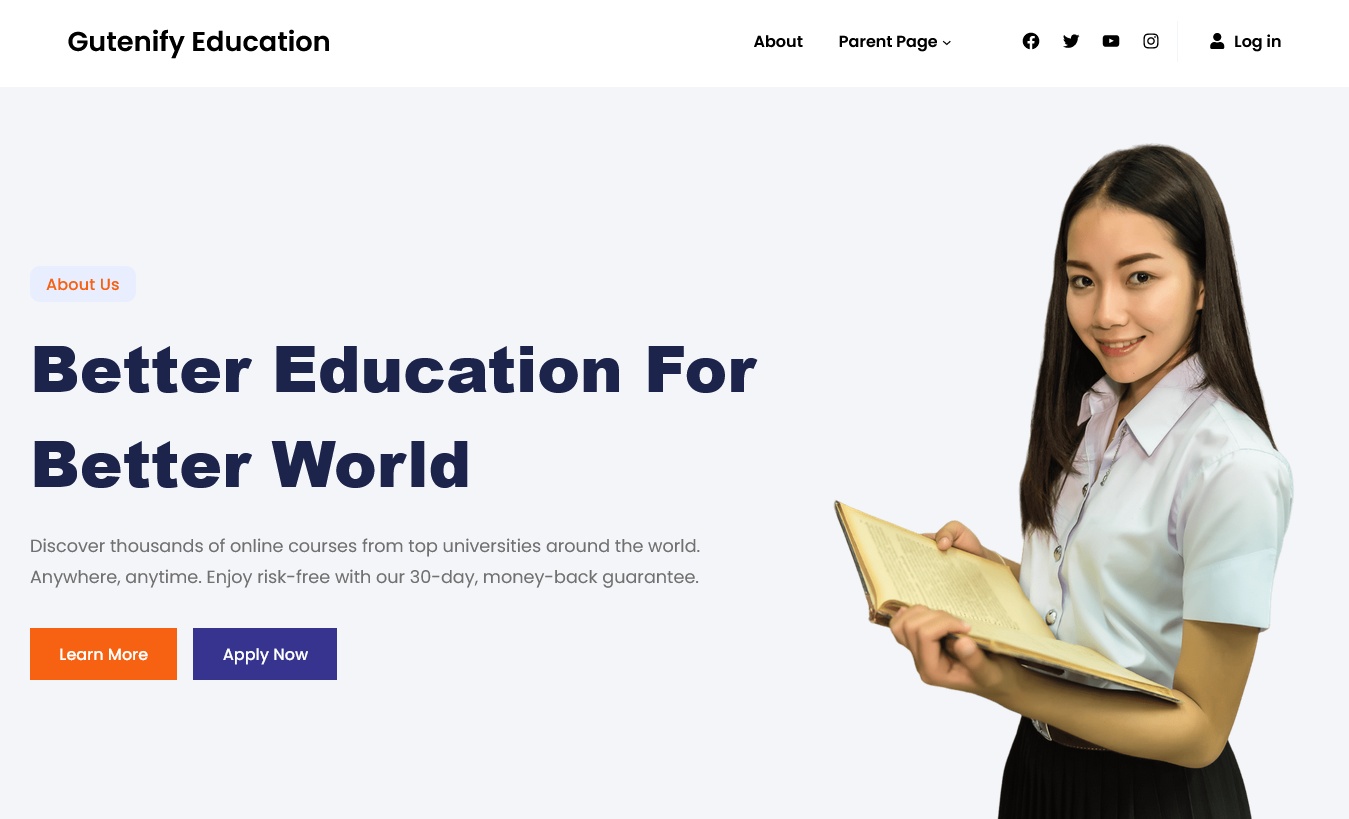The image, captured as a horizontally rectangular screenshot from a website, features a clean and organized layout with distinct elements. 

At the top, there is a white banner displaying the title "GUTENIFY EDUCATION" on the left. The title is spelled out as G-U-T-E-N-I-F-Y. On the right, just off-center, the banner contains navigation options including "About," "Parent Page," and icons for social media platforms such as Facebook, Twitter, YouTube, and Instagram, alongside a login icon.

Below the banner, the background transitions to a light gray. The focal point is a woman with long black hair, standing slightly sideways but facing left towards the viewer. She is smiling warmly, dressed in a white short-sleeved, button-up collared shirt, and holding an open book. 

To the left of the woman is an "About Us" link button. Directly below, in large bold font, the slogan "Better Education for Better World" is prominently displayed. Beneath this tagline, in a standard-sized font, is the description: "Discover thousands of online courses from top universities around the world. Anywhere, anytime, enjoy risk-free with our 30-day money-back guarantee."

At the bottom left of this section, there are two call-to-action buttons side-by-side: an orange button labeled "Learn More" and a blue button labeled "Apply Now."